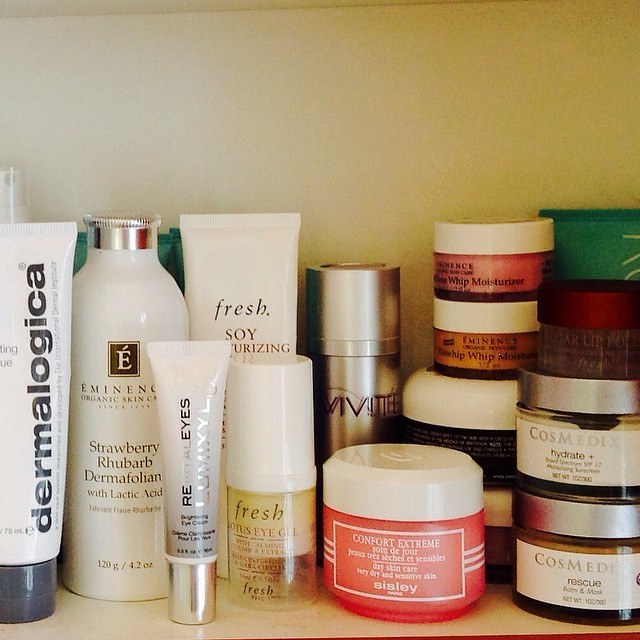A neatly arranged collection of various skin care products is displayed on a pristine white shelf. The softly illuminated background features a gentle whitish-yellow hue, providing a warm contrast to the array of items. On the far left, there is a white tube of Dermalogica product, distinguished by its vertical dark gray lettering and matching gray cap. Adjacent to this, moving rightward, sits a white bottle labeled "Strawberry Rhubarb Dermafoliant with Lactic Acid" from Eminence.

In front of the Eminence bottle, there's a petite tube of eye cream capped with a striking silver top. Directly behind it stands another white tube, marked "Fresh Soy Moisturizing." Complementing this, positioned closer to the viewer, is a small bottle of "Fresh Eye Gel," easily identifiable by its substantial white cap.

Further right along the shelf, a distinctive collection of jars can be seen, prominently featuring the "Comfort Extreme" range by Sisley. Each jar, either red or pink in hue with a contrasting white cap, stands neatly in line, adding a touch of vibrant color to the arrangement. In total, eight jars of miscellaneous skin care brands are methodically placed to the far right, completing this meticulously organized display.